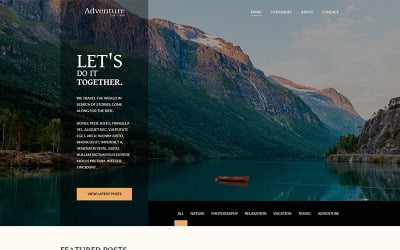Screenshot of a Website Promoting Adventure Trips:

The image captures a website with a scenic background featuring a majestic landscape of mountains and a serene lake, in the center of which floats a vibrant orange-red boat. Overlaid on this picturesque scene is a mostly opaque black box, contrasted with white text. At the top of the box, the word "Adventure" is prominently displayed, followed by the phrase "Let's do it together." Additional text, which appears blurred and unreadable, is situated below this tagline.

Towards the bottom of the overlay, a coral-colored button suggests a call to action, likely allowing users to engage further with the site. Along the top navigation bar, various menu options are listed, although their titles remain unclear due to the resolution. These options are presumably standard categories such as "Home" and "About."

At the bottom of the page, another black box with white text is present, which is similarly unreadable. The leftmost option among the seven clickable sections on this nav bar is highlighted with an orange box, indicating that it is the current selection.

Overall, this screenshot appears to be from a website dedicated to organizing or promoting adventure trips, offering picturesque visuals and accessible navigation options to attract and assist potential adventurers.